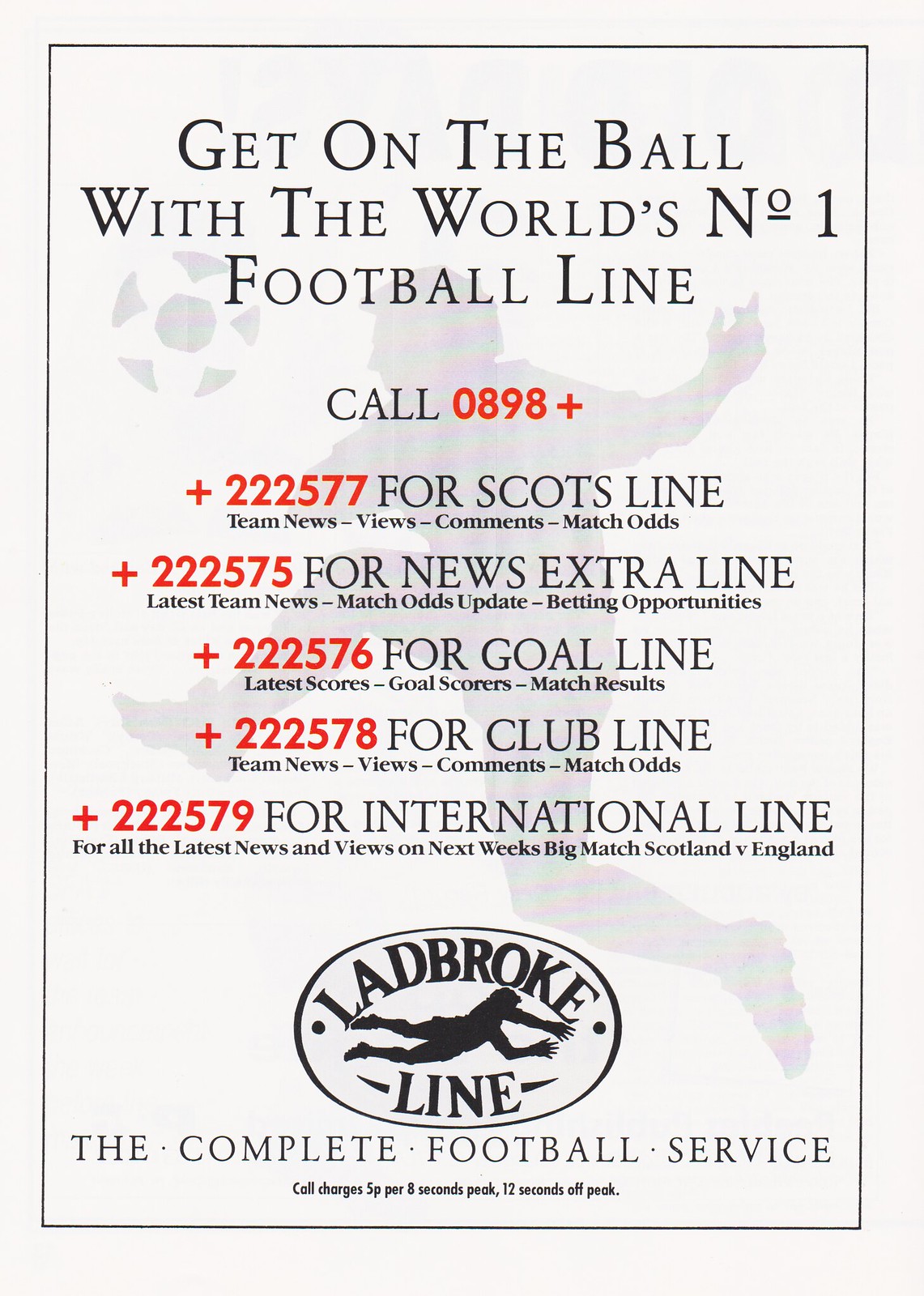The image is a full-page advertisement from an old magazine, featuring a black, white, and red color scheme. At the center, large text reads, "Get on the Ball with the World's Number One Football Line." Behind the text, a football player is seen mid-jump, his right leg raised towards his chest while his left leg is bent back—a soccer ball is approaching his chest from the left. 

Prominent red text instructs readers to "Call 0898 Plus" followed by various specialized lines for detailed football updates:
- **Scott's Line**: +222577 for team news, views, comments, and match odds.
- **News Extra Line**: +222575 for the latest team news, match odds updates, and betting opportunities.
- **Goal Line**: +222576 for the latest scores, goal scorers, and match results.
- **Club Line**: +222578 for team news, views, comments, and match odds.
- **International Line**: +222579 for the latest news and views on next week's big match, Scotland vs. England.

At the bottom, the logo reads "Ladbroke Line" with the tagline "The Complete Football Service." Call charges are specified as 5p per 8 seconds during peak times and 12 seconds off-peak.

Overall, the ad promotes a football information service with various lines dedicated to different aspects of the game, emphasizing its comprehensive coverage and the ongoing rivalry between Scotland and England.